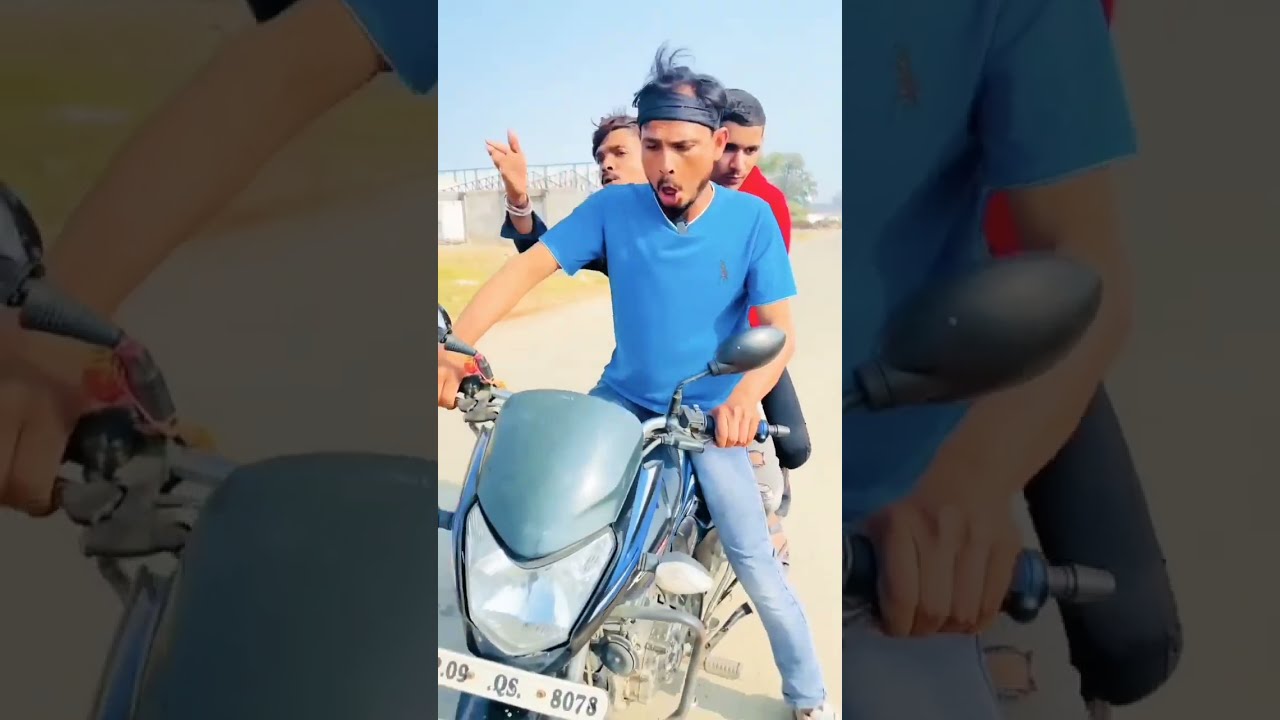In this lively image, three men in their 20s are riding a somewhat old and not very large blue motorcycle, appearing to perform a stunt on a sunny day. The rider at the front is wearing a blue shirt with a black logo on the left side, blue jeans, and a black headband wrapped around his medium-length black hair. His mustached face displays an expression of exhilaration as he screams, likely fueled by adrenaline. Behind him, a man in a red shirt and black pants sits, though his position on the bike is unclear. The third man in the back wears a long-sleeved black shirt and a white bracelet on his wrist. He is holding up his hand in a gesture, possibly to maintain his balance or adding to the stunt's drama. Their combined energy and the clear outdoor setting amplify the adventurous spirit of the moment.